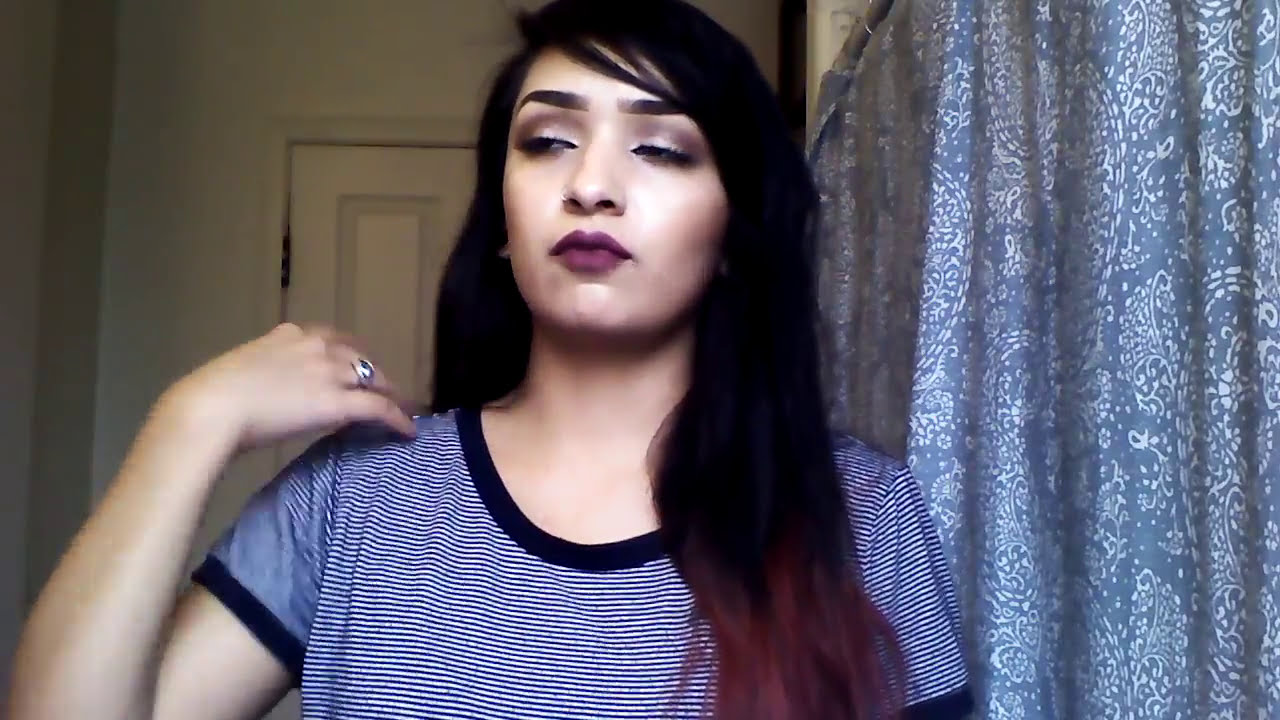This photograph captures a woman with long, dark hair that has purple tips. She is wearing heavy purple eyeshadow, matching her purple lipstick. Her attire consists of a black and white striped t-shirt with blue borders on the sleeves and neckline. The woman is sitting in what appears to be a bathroom, with a closed white door and a blue and white shower curtain or window curtain hanging from a white wall behind her on the left. She is looking slightly to her right with her eyes partially closed, and her right hand is raised, touching her shoulder. On her right hand, she wears a silver ring, adding a touch of detail to her poised, yet candid demeanor.